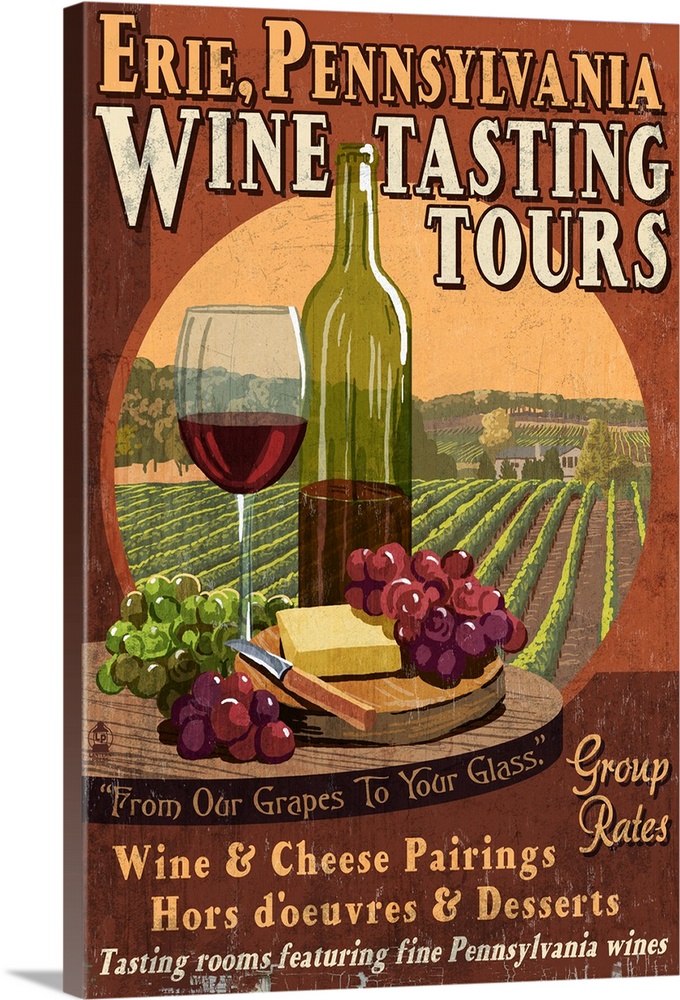An advertisement, likely a book cover or promotional poster for Erie, Pennsylvania Wine Tasting Tours, features a rich rust-burgundy background. The centerpiece displays an illustrated or photographed winery landscape, with lush rows of grapevines stretching endlessly into the distance. In the foreground sits a detailed still life: a round wooden cutting board laden with a half-full green bottle of burgundy wine, a matching half-full wine glass, green and red grape clusters, a block of cheese, and a knife. Prominently displayed text includes "Erie, Pennsylvania" at the top in orange, and beneath it, "Wine Tasting Tours" in white. Additional text at the bottom reads, "From Our Grapes to Your Glass - Group Rates, Wine and Cheese Pairings, Hors d'oeuvres and Desserts - Tasting Rooms Featuring Fine Pennsylvania Wines."